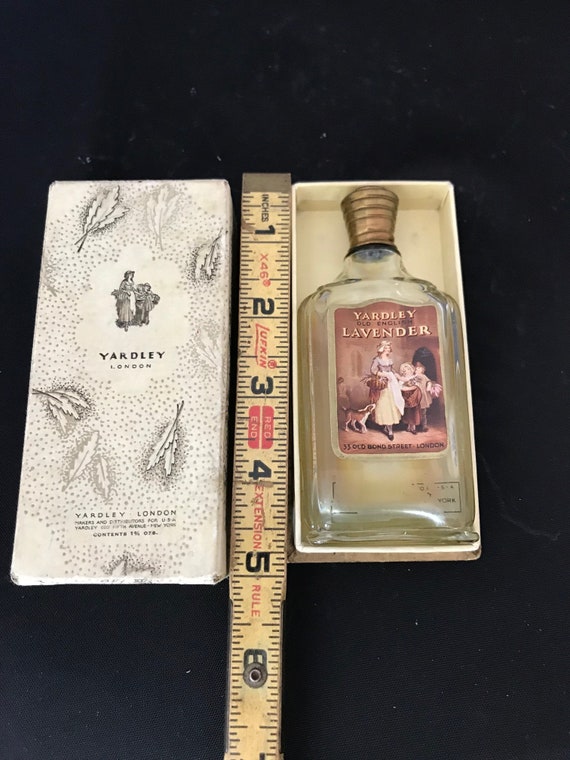The image depicts a vintage Yardley Lavender bottle, housed within a white cardboard box adorned with depictions of lavender leaves and the text "Yardley London" on the top. The bottle itself is made of clear glass and has a brass screw-on cap, bearing a label that reads "Yardley Lavender" and includes "33 Old Bond Street, London" at the bottom. The box's dimensions are highlighted by an adjacent tape measure, showing it to be just under five inches in length. Initially mistaken by some viewers for a liquor bottle due to its shape, the detailed floral and text elements strongly suggest it is a historical perfume bottle, likely used by women in the past.